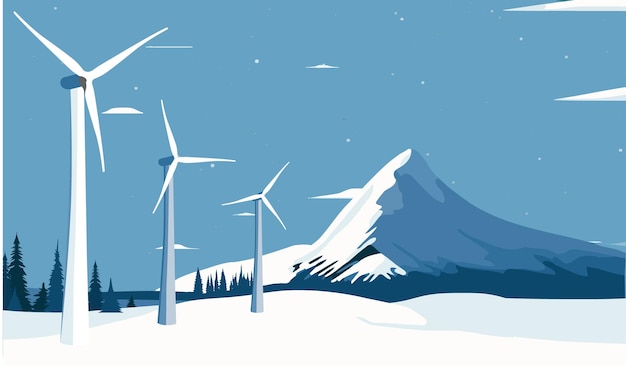The image is a stylized, horizontal illustration with a predominant blue background, featuring a snowy landscape. In the foreground are three modern windmills with three blades each, positioned in a diagonal row from left to right. They stand tall amidst a ground blanketed with piles of snow. To the left and lower corner of the image, there are tall evergreen trees, adding a touch of green to the predominantly white and blue scene. The sky above is light blue, dotted with small, distant, white clouds and white specks suggesting snowfall or a starry night. In the far background, there is a majestic mountain covered in snow, with a prominent peak rising high. The overall composition, with its serene pastel colors and wintery elements, gives the impression of a tranquil, snowy setting often seen on postcards.